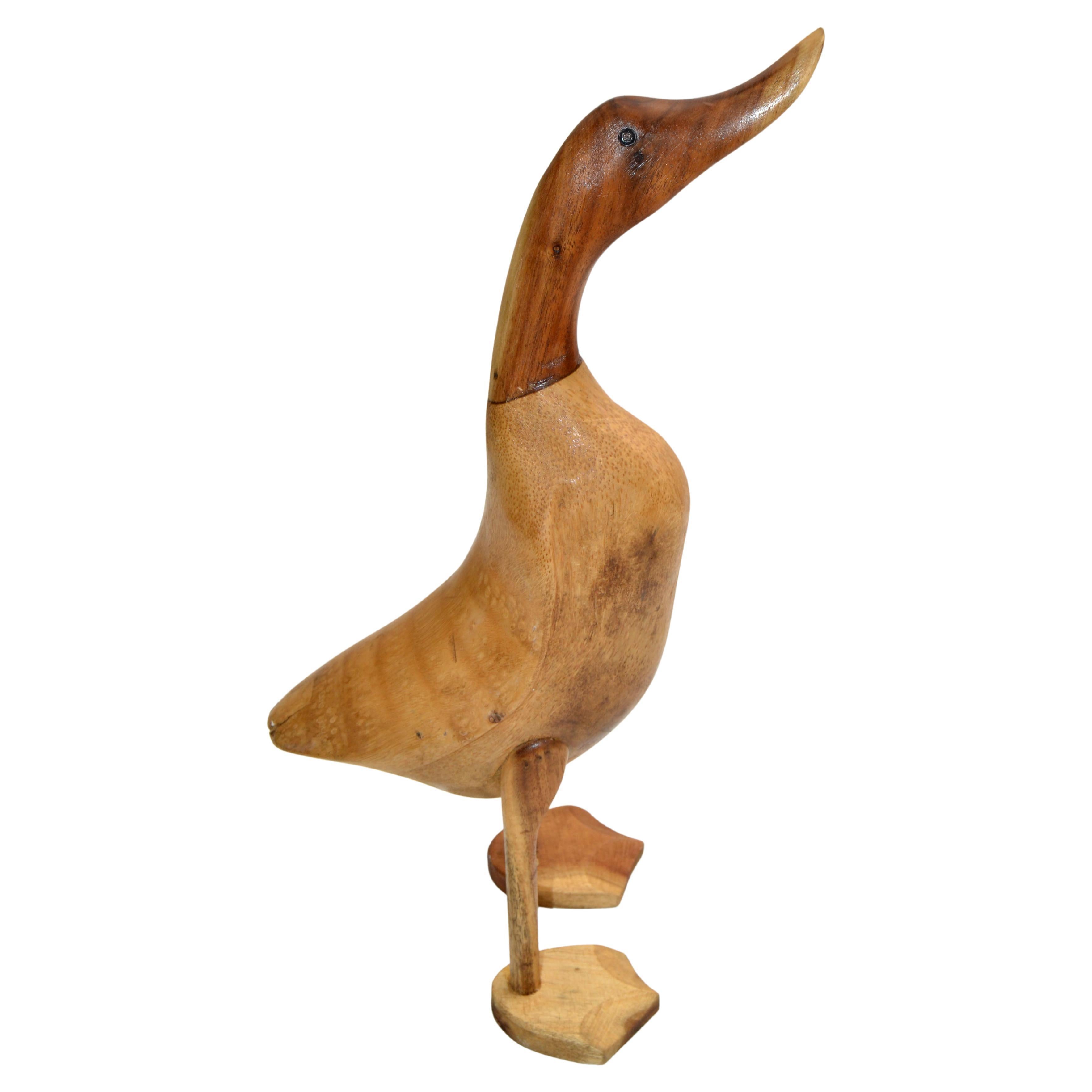This image depicts a meticulously carved wooden duck, showcased on a light, unadorned background that allows the intricate details to stand out. The duck is carved in a profile pose, facing the left, with its elongated neck stretched upwards and its beak pointed towards the sky. The head and neck of the duck are crafted from a darker, polished wood, possibly with an orangey stain, adding a touch of elegance to its graceful posture. Transitioning from the neck to the body, the wood becomes lighter, perhaps maple, adorned with subtle darker spots that add to its rustic charm. The body itself is elongated, flowing seamlessly into the lighter wood. The duck stands on two spindly wooden dowels, about half an inch in diameter, which serve as its legs, ending in flat, handcrafted duck feet. The overall appearance suggests it could be a woodworker's creation, ideal as a decorative item in a country-style home or potentially even as a hunting decoy. The absence of wings and the handcrafted aesthetic further highlight its unique, artisanal quality.